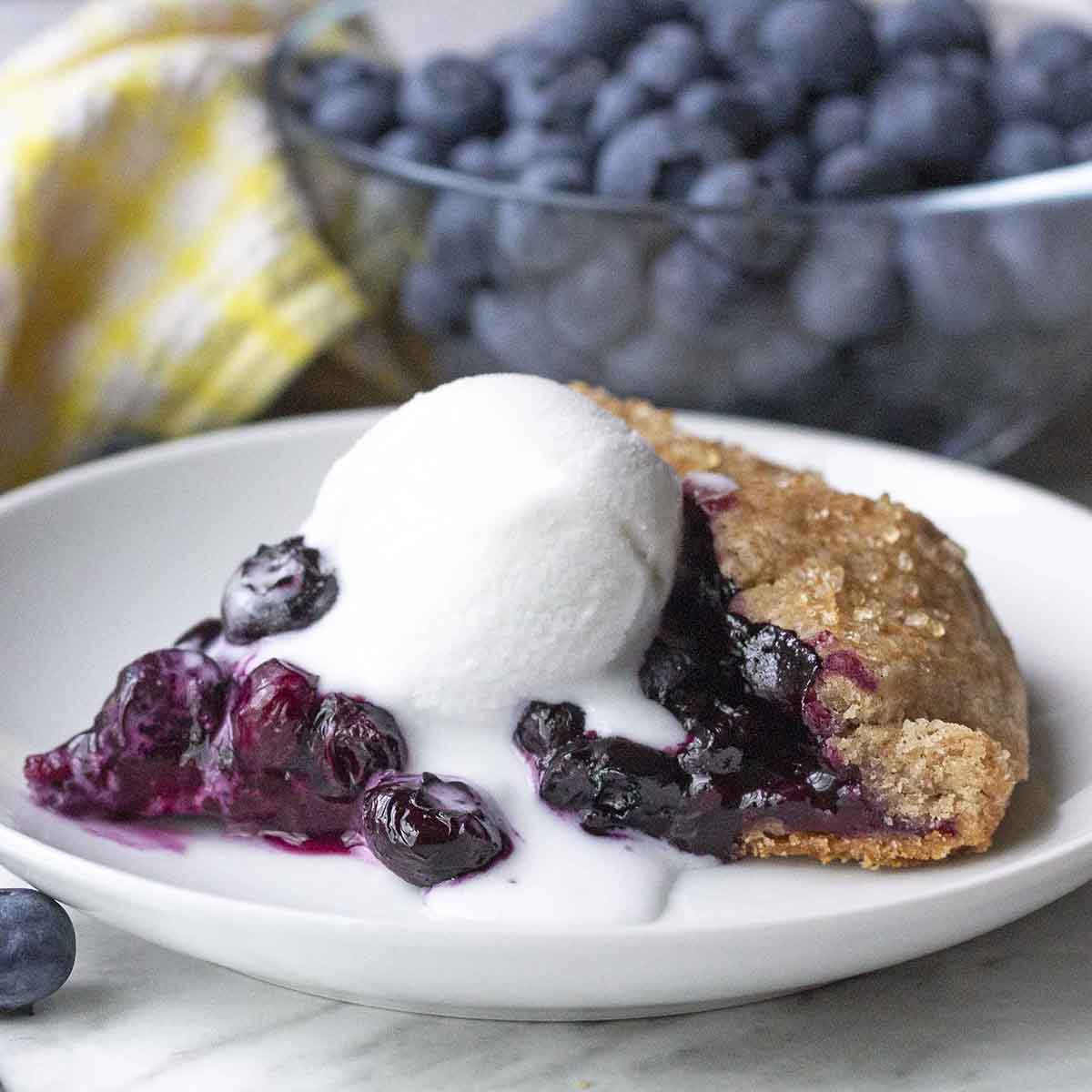The image showcases a delectable blueberry cobbler set on a circular white ceramic plate, resting atop a gray and white marble tabletop. The cobbler boasts a golden brown crust with a dusting of sugar crystals, and it's topped with a generous scoop of vanilla ice cream beginning to melt slightly. In the background, there's a clear glass bowl brimming with fresh blueberries and a white and yellow plaid kitchen towel to the left. One solitary blueberry sits at the bottom left of the image on the marble counter. The focus is sharply on the front, highlighting the dessert's textures and colors vividly, while the background elements remain softly blurred, enriching the vibrant and inviting presentation of the scene.